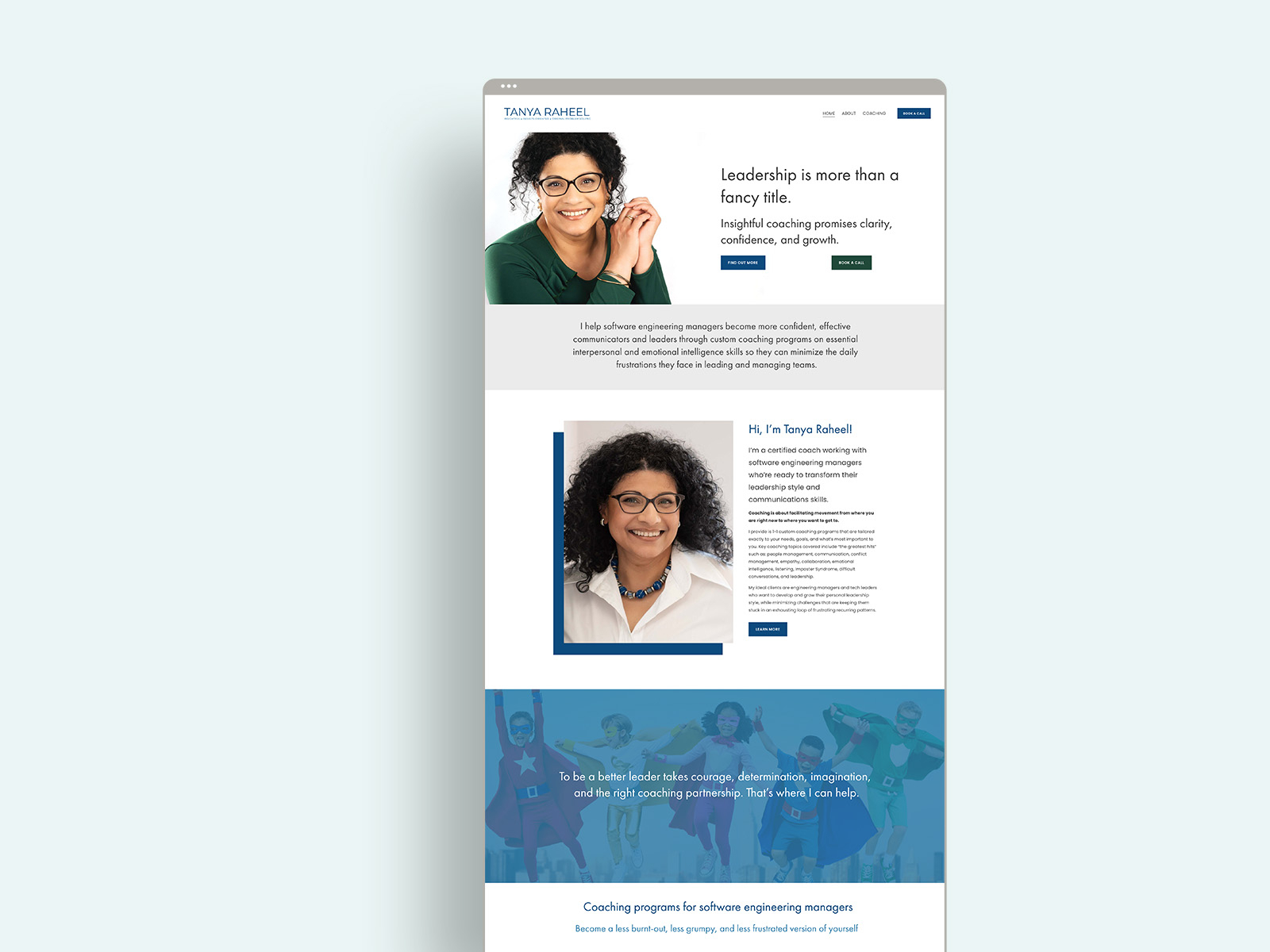The image showcases a website for Tanya Rahel. The background features a faint aqua-blue color. The site appears to be displayed on an Apple device, indicated by a subtle shadow on the left-hand side. The heading "Tanya Rahel" is prominently displayed and underlined.

The website contains a profile section with a headshot of Tanya, a woman in her mid-30s to early 40s, wearing glasses and a green long-sleeved shirt. She has black, curly hair styled up. Accompanying the picture, there's a motivational quote: "Leadership is more than a fancy title," followed by a paragraph that is not fully legible from this view. Below this section, there are two buttons—one green and one blue—set on a light gray banner.

Further down, another photograph of Tanya is displayed where she's smiling, wearing a different outfit, and a necklace. Her hair is slightly down in this image. The accompanying text starts with, "Hi, I'm Tanya Rahel," followed by a body paragraph and a blue button below.

Towards the bottom of the page, there is an image of children wearing capes overlaid with centered text that offers additional information. The overall design of the website is clean and engaging, highlighting Tanya Rahel’s professional and motivational persona.